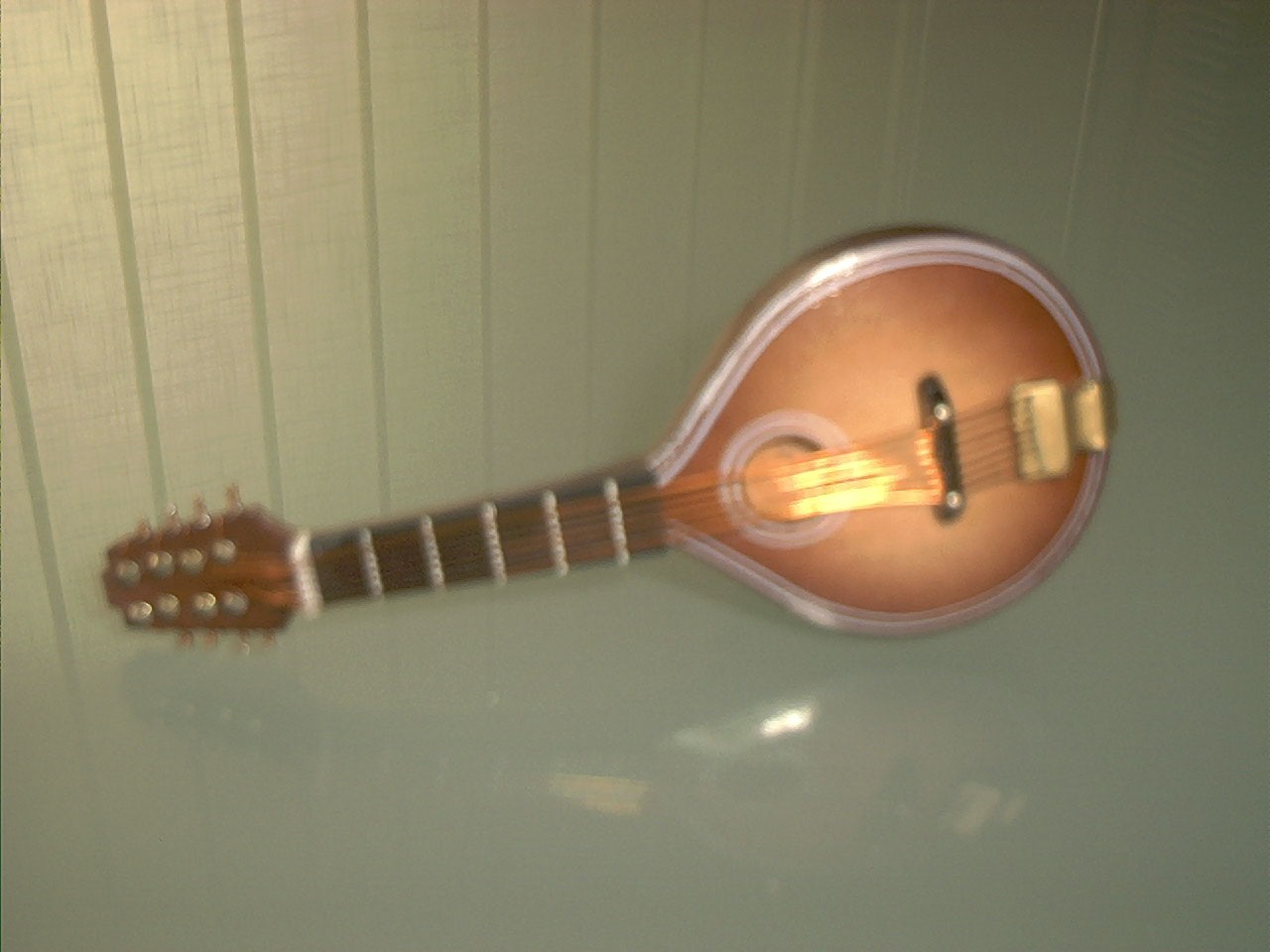In the image, there appears to be a blurry photograph of a banjo laying on its side on a polished white surface, with a pale greenish backdrop, which could either be a wall or a table. The banjo itself has a circular body on the right side, bordered with a white trim, while the neck extends to the left, featuring dark brown frets. The face of the banjo, which holds the strings, is lighter brown and appears to have gold-colored strings facing the viewer. The instrument looks shiny and new, without visible signs of wear. The polished surface catches a slight reflection of the banjo, adding a touch of visual depth to the image despite the blurriness.